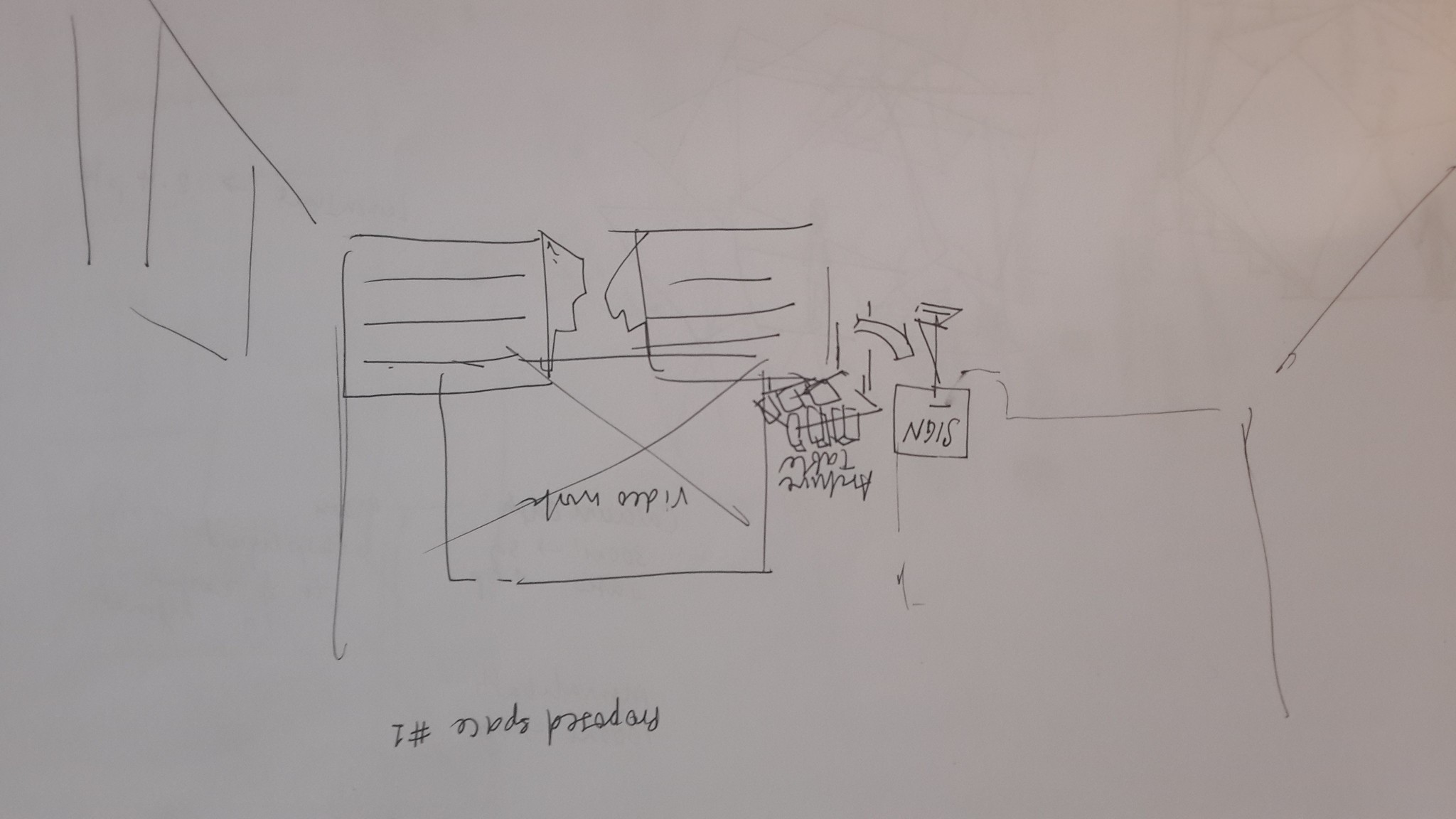This is a hand-drawn, albeit hastily and poorly done, pencil sketch that appears to be a proposal update, labeled "Proposed Update Number One." The entire image is upside down, making it difficult to interpret accurately. In the drawing, there is an 'X' marked on some video work, a sign, and a table that seemingly holds bottled water. The sketch also depicts two desks with lines drawn to indicate details, and the walls and floor of a room. Additionally, the paper shows signs of other drawings from the opposite side, with pencil marks and faint images bleeding through. The paper itself is a grayish-white hue, evidencing numerous erasures and corrections. Unfortunately, the purpose behind this proposal remains unclear due to the lack of context and the ambiguous depiction.